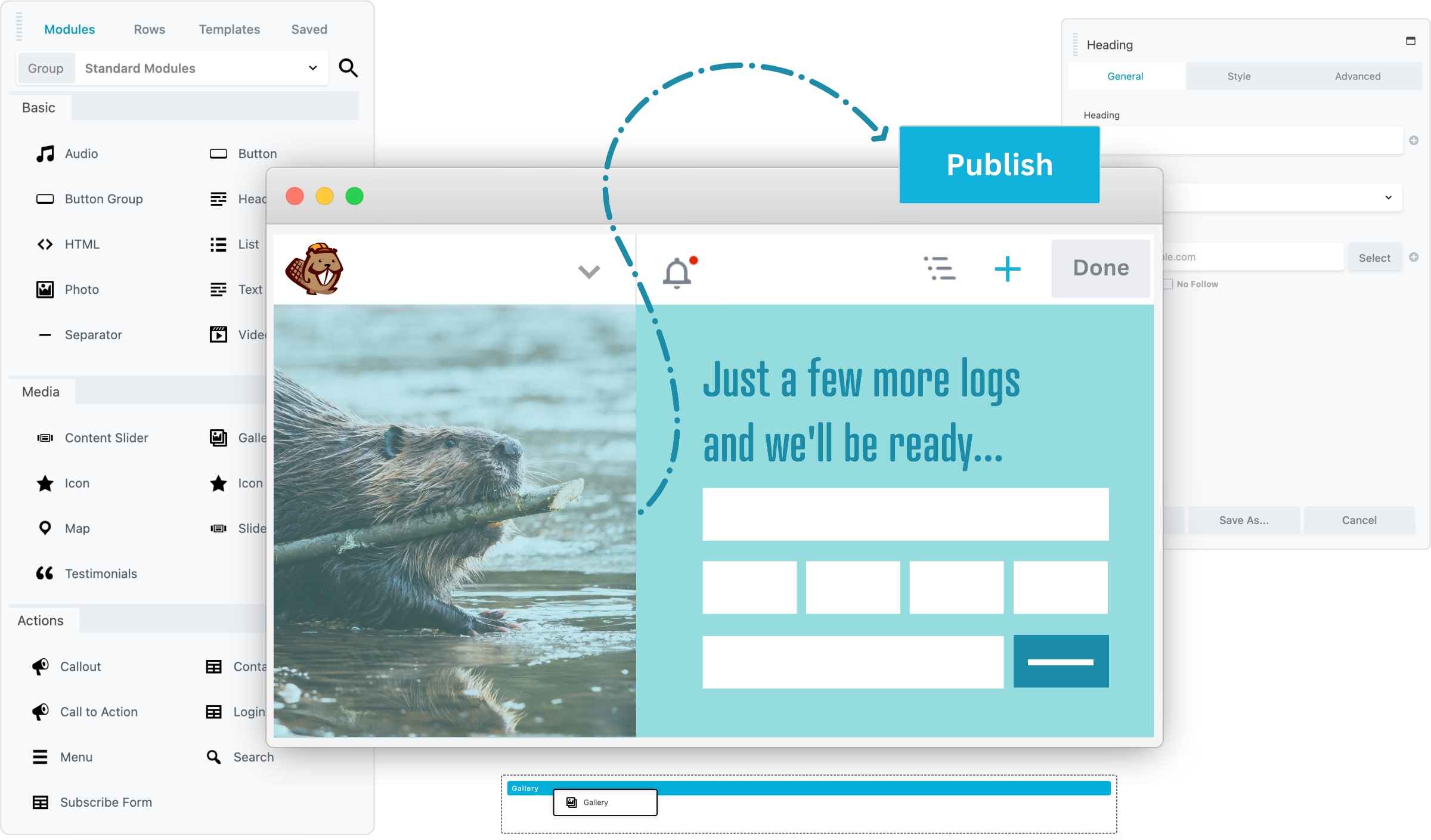The left side of the interface features a menu at the top that includes four tabs: Modules, Rows, Templates, and Saved. Beneath this menu is a search bar labeled "Standard Modules." Directly under the search bar, there are categorized sections titled Basic, Media, and Action, each containing various items. The interface itself is divided into two columns on the left side. The left column lists options such as Audio, Button Group, HTML, Photo, Separator, Content Slider, Icon, Map, Testimonials, Callout, Call to Action, Menu, and Subscribe Form. The contents of the right column are obscured by a pop-up.

The pop-up displays a picture of a beaver, a notification icon, and a cartoon image of a beaver. It includes a gray 'Done' button and a light blue square containing dark blue text that reads, "Just a few more logs and we'll be ready." Below this text are six white input boxes for user information. In the bottom right corner of the pop-up is a dark blue box.